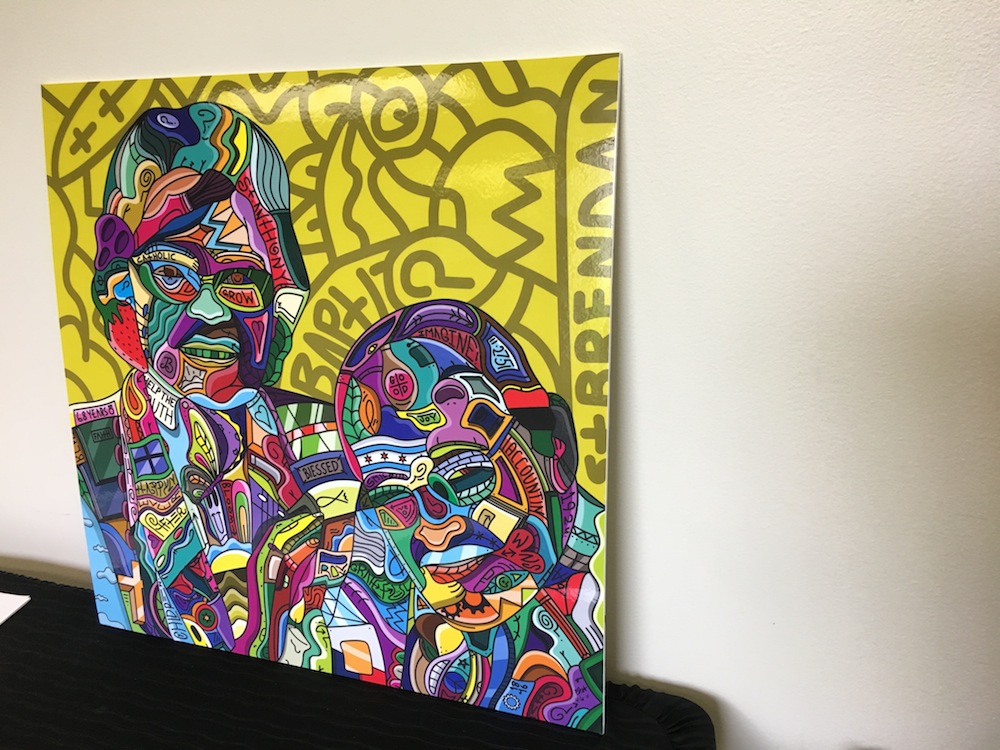The image displays an abstract, psychedelic poster featuring two multicolored figures positioned in front of a vibrant yellow background with brown text that reads "St. Brendan." The poster also incorporates the word "Catholic" over one figure's eye and "crow" below the same eye. Additionally, there are various other words scattered throughout the design, including "help," "grow," "the truth," and "joy." Both figures are composed of an eclectic mix of shapes, colors, and imagery such as red, orange, green, and blue patches, eyeglasses, lips, question marks, and fish. The figures appear to be seated on a black table, and the yellow background includes two plus-shaped decorations. The letters "B-A-P-T-I-Z" are depicted above a bird within the intricate background, contributing to the captivating, enigmatic quality of the artwork.